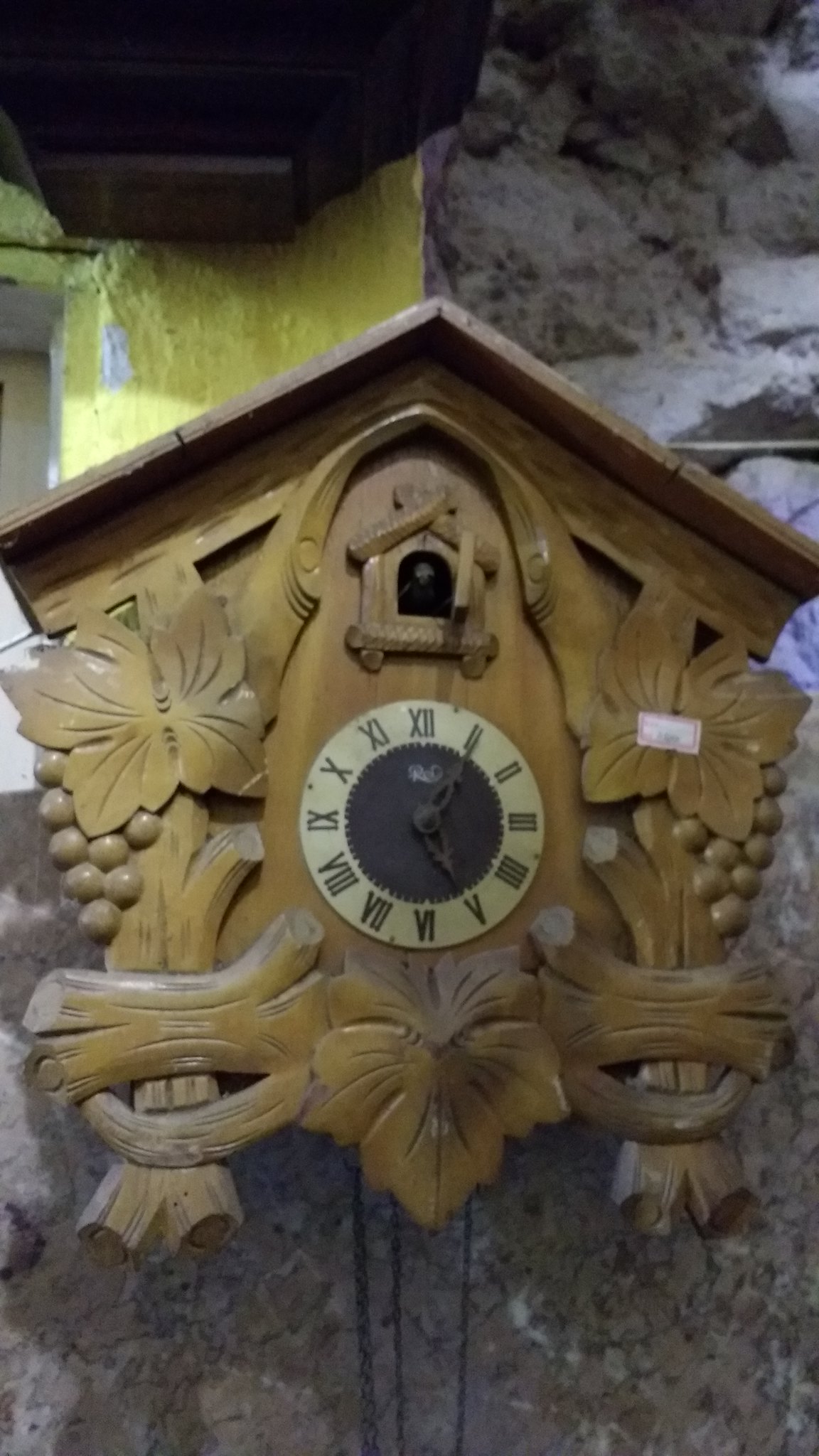This image features a detailed photograph of a hand-carved, antique wooden cuckoo clock hanging on a rustic gray stone wall. The clock, primarily brown, showcases an intricately designed exterior with various decorative elements including butterflies and clusters of grapes symmetrically placed on both the left and right sides. The bottom left and right sections feature log-like shapes. At the top, a smaller birdhouse-shaped structure houses a mini door, which is open, revealing a cuckoo bird emerging mid-squawk. The clock's face prominently displays Roman numerals, with a border that transitions from white on the outer ring to black in the center. Three strings, likely tied to chimes, hang down the middle, hinting at the clock's capability to chime. A subtle white sticker is present on the right, adding to the details. The time on the clock reads 2:40. The craftsmanship, combining elements of nature and antique design, highlights the clock's wooden flowers, leaves, and potentially berries or grapes, making it a unique and decorative piece.